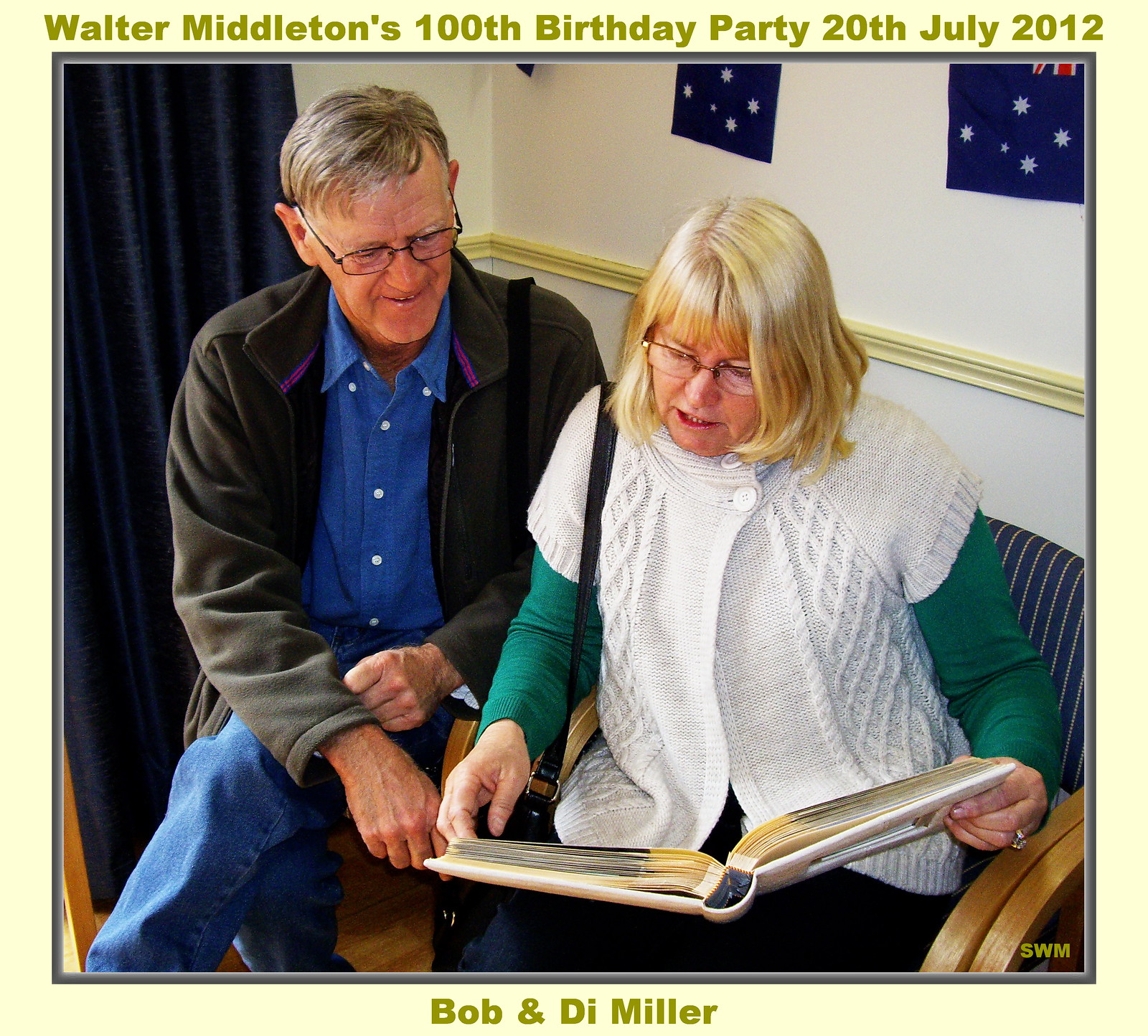This photograph, framed in gray against a pastel yellow background, captures a moment from Walter Middleton's 100th birthday party on 20th July 2012, as noted in dark yellow font above the image. The central focus is an older couple, Bob and Dee Miller, seated and engaged in looking at a scrapbook or photo book. Bob, situated on the left, sports glasses, jeans, and a button-down shirt layered with a light jacket. Dee, on the right, wears glasses, has short blonde hair, and is dressed in green sleeves with a white knit sweater. Behind them, the white wall is adorned with small British flags, and blue curtains are visible to the back left of the photograph.